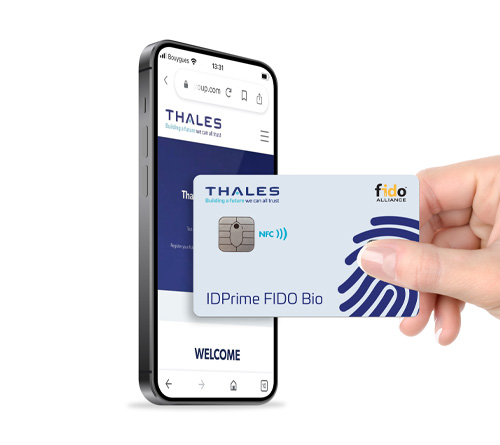A close-up image showcases a female hand holding a light blue Thales ID Prime FIDO Bio credit card against a white backdrop. The hand's thumb and forefinger grip the card, which is prominently displayed. The card features blue writing on the top left that reads "Thales," with additional text below that says "ID Prime FIDO Bio." A blue fingerprint icon is on the right side of the card, while the top right displays the FIDO Alliance logo in black and yellow. The card includes an NFC chip on the left side.

The credit card is being tapped against a gray Apple smartphone, which is showing the Thales website—a sign-in page with white and blue accents. The website includes a welcome message and a search bar at the top, indicating this might be a secure payment or authentication process. Both the card and the phone suggest a secure, advanced biometric and NFC-enabled financial transaction.